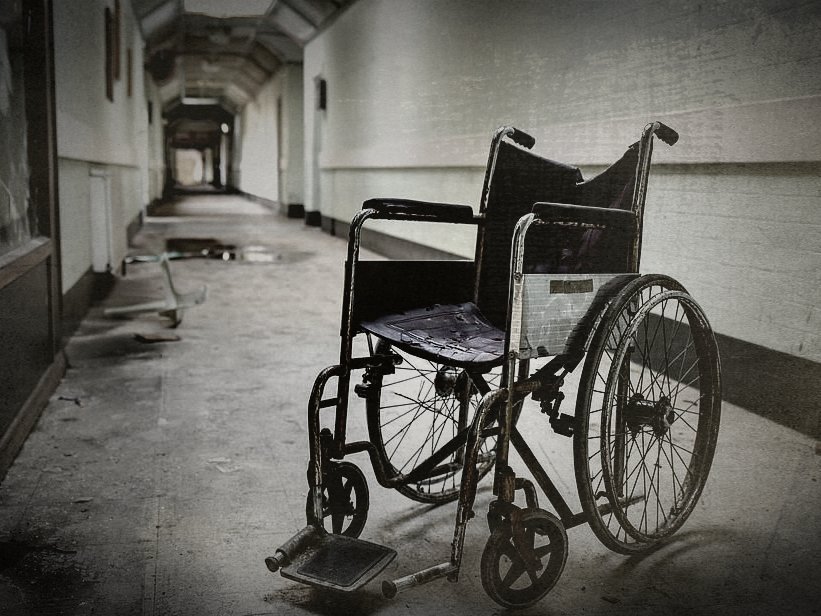The black-and-white photograph captures a long, arched hallway that appears abandoned and currently unused. The floor is littered with droplets and patches of water, as well as scattered papers, indicating neglect and a lack of recent human activity. Dominating the foreground is a damaged, empty wheelchair facing toward the lower left corner of the image. The wheelchair has several missing or broken pieces: its left footrest is partially missing, the tires appear deflated, and the leather seat is torn and bent, possibly suggesting long-term disrepair. The hall's flooring is also in poor condition, with sections coming up on the left side and a notable pothole in the middle of the path. The walls feature a darker trim running along the bottom, adding to the overall desolate and worn-out atmosphere of the scene.